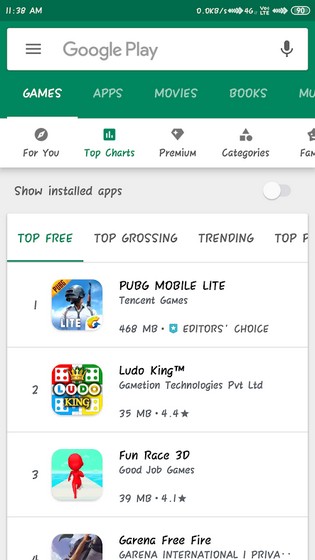**Detailed Image Description: Google Play Store Browsing**

The image captures a screenshot of a mobile phone in portrait orientation displaying the Google Play Store app. The top status bar reveals the phone's details: at 11:38 AM, with a data speed indicator showing "0.0 kb/s," followed by a series of network status icons—five arrows (signal strength), "4G," "WE" with "LTE" below, the five arrows again, and a battery symbol indicating 90% charge.

Below this status bar is a white search bar spanning the width of the screen, featuring three gray horizontal lines (menu icon) on the left, the text "Google Play" in gray in the center, and a microphone icon on the right. The search bar is overlaid on a green navigation banner that contains the tabs: "Games," "Apps," "Movies," "Books," and "Music" in white lettering, with the "Games" tab highlighted.

Directly under this green banner, there is a secondary navigation bar for the "Games" tab with options: "For You," "Top Charts," "Premium," "Categories," and "Familiar" or "Favourites." Below this, a prompt reads "Show Installed Apps" with a white toggle button on the right.

The main content area of the screen is a white table with the tabs "Top Free" (highlighted in green), "Top Grossing," "Trending," and an unreadable tab, which extends out of the viewable screen area. The visible portion lists the top four free games:

1. **PUBG Mobile Lite**: Displaying the icon for PUBG Mobile Lite by Tencent Games, marked with "Editor's Choice" and sized 468MB.
  
2. **Ludo King**: Featuring a logo with colorful letters—L (blue), U (red), D (green), O (yellow)—each on white backgrounds. Surrounding the letters are dice icons:
   - Top-left: White dice with four red dots on a red background.
   - Top-right: White square with four green dots on a green background.
   - Bottom-left: White square with four blue dots on a blue background.
   - Bottom-right: White square with four yellow dots on a yellow background.
   The text "Ludo King" is adorned with a crown above "Ludo" and "King" written in gold below it. Created by Gametion Technologies Pvt. Ltd., the game occupies 35MB and has a 4.4-star rating.
   
3. **Thunrace 3D**: Showing a red figure running on a concrete runway with a green sky background, accompanied by the text "Thunrace 3D," developed by Good Job Games, occupying 39MB and rated 4.1 stars.
   
4. **Garena Free Fire**: Only partially visible, displaying the text "Garena Free Fire" by Garena International. The logo is obscure and difficult to identify.

This detailed description captures the intricate visible elements and interface specifics of the Google Play Store as displayed on a mobile device.